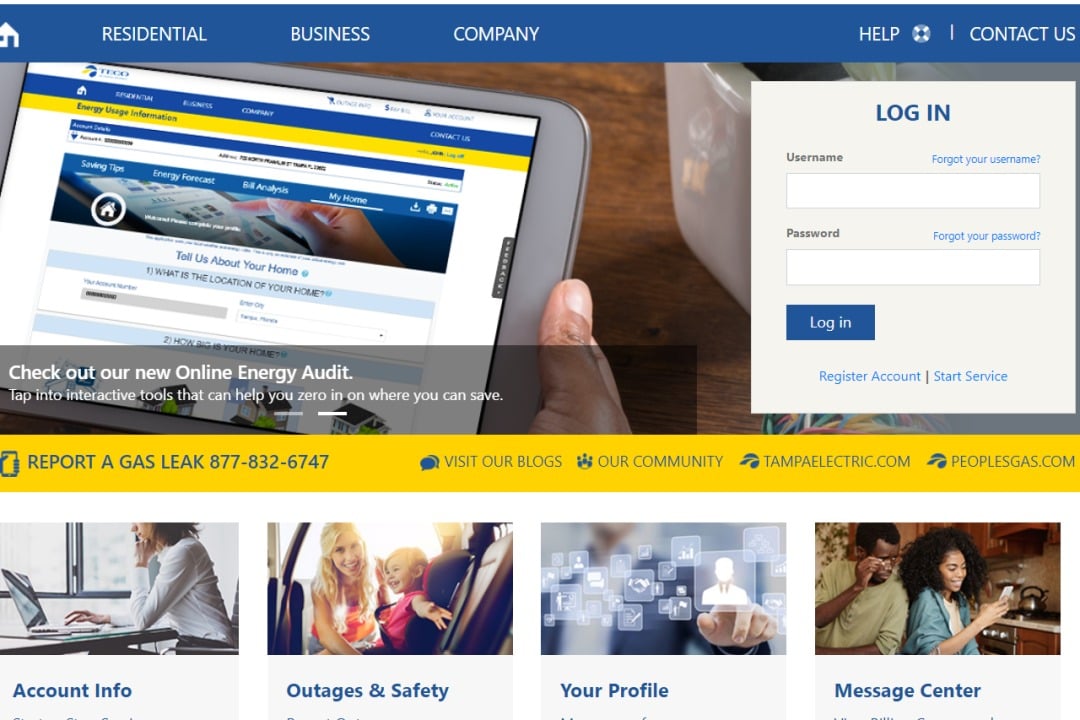This image is a color screenshot from an unknown website, featuring a comprehensive layout aimed at providing various services and information to users. At the top, a blue banner displays navigation options in white lettering: "Residential," "Business," "Company," "Help," and "Contact Us." An image shows a person's right thumb and fingers holding a tablet sideways, which displays a screenshot of the same webpage.

Below this, there is a highlighted message promoting their new online energy audit, encouraging users to tap into interactive tools for energy-saving insights. Important contact information is provided for reporting a gas leak (877-832-6747) and links to visit their blogs, community pages, and two related websites: tampaelectric.com and peoplesgas.com.

In the top right corner, a white box facilitates user login, offering fields and links for logging in, username and password recovery, new account registration, and starting a service. 

Further down the page, different service categories are illustrated:

1. **Account Info:** Accompanied by an image of a person at a desk using a laptop.
2. **Outages and Safety:** Featuring a woman securing a smiling child into a car seat.
3. **Your Profile:** Displaying several small icons with white images.
4. **Message Center:** Depicted with an image of two African American individuals, where a man looks over his glasses at a smartphone held by a woman.